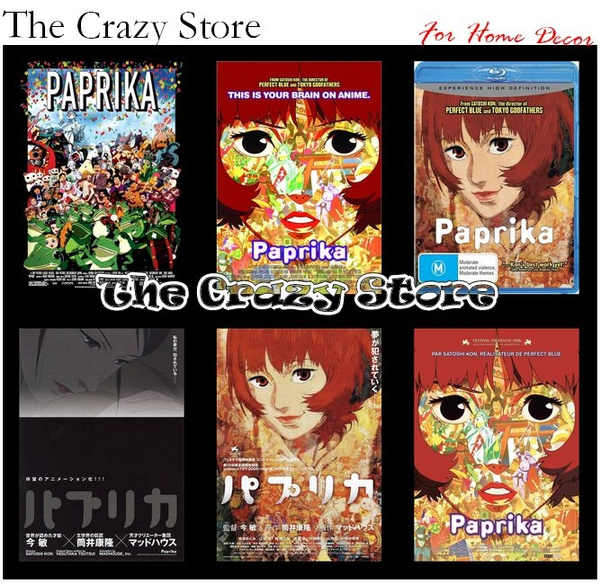The image is a detailed collage showcasing six different Blu-ray covers for the anime movie "Paprika," prominently featuring a woman with jaw-length red hair and striking black eyes. The collection is visually vibrant, with each cover highlighting different artistic styles. In the top left, one cover is filled with a crowd of characters and distinct artistic flair, accompanied by the phrase "The Crazy Store." The top middle cover declares "This is your brain on anime," presenting a woman's face composed of an intricate collage of images. This same face, with her expressive features and red hair, appears on multiple covers. The top right and bottom right covers share a similar design, both with a black background emphasizing the Blu-ray format. Meanwhile, the bottom left cover is in black and white, displaying only Asian script. In the center of the entire image, the text "The Crazy Store" appears again, suggesting an ad or promotion, potentially for home decor. Detailed and colorful, the image captures the diverse visual representations of the film "Paprika" in an anime style.